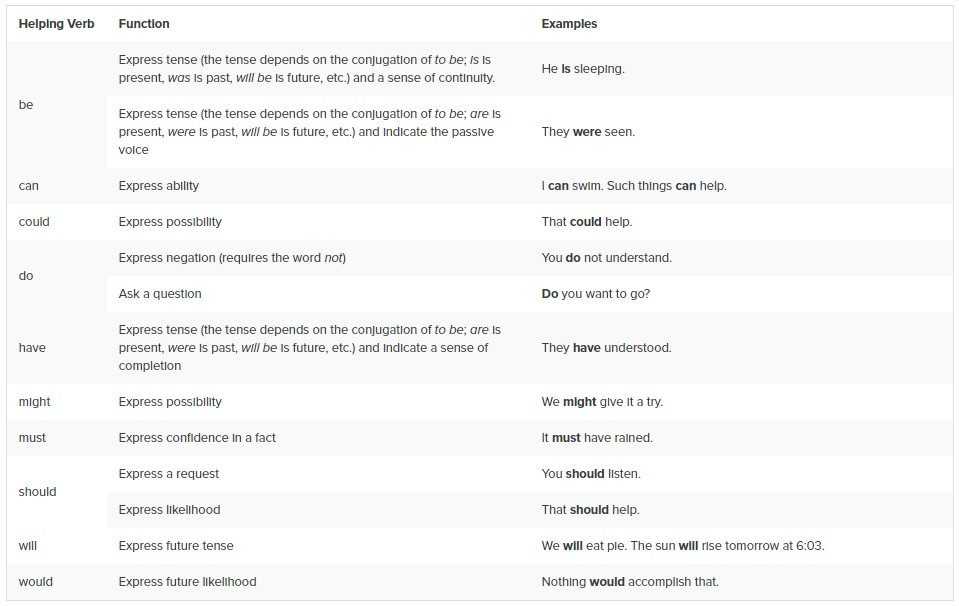Image Description: A Detailed Guide to Helping Verbs and Their Uses

This meticulously organized image serves as a comprehensive guide to various helping verbs. The entire layout is presented on a striped background of light gray and white, giving it a clean and structured appearance, while the informational text is rendered in bold black for clarity.

The content is systematically arranged into three columns labeled from left to right as follows: "Helping Verb," "Function," and "Examples." The helping verbs listed in the first column include: "be," "can," "could," "do," "have," "might," "must," "should," "will," and "would."

In the "Function" column, detailed information is provided about what each helping verb expresses. This explanatory text offers a precise description of the grammatical and semantic role that each helping verb plays within a sentence.

Finally, the "Examples" column to the right demonstrates the use of each helping verb in context. Each example sentence has the pertinent helping verb highlighted in bold, making it easy to identify within the sentence, while the remaining text of each example remains in regular font.

This image serves as an invaluable resource for understanding the purpose and application of helping verbs, effectively bridging the gap between theoretical grammar knowledge and practical usage.